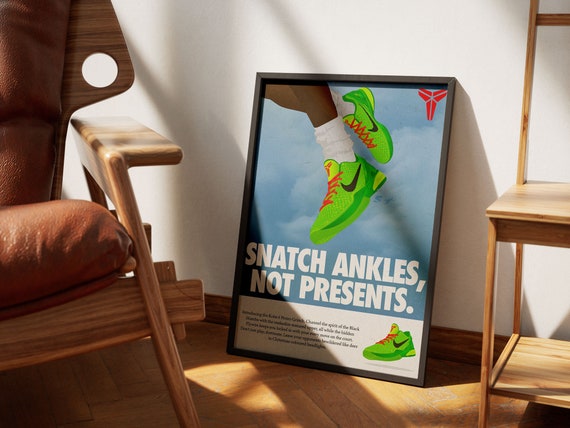This detailed color photograph captures an indoor scene featuring sleek, mid-century modern furnishings against a minimalist backdrop. At the bottom, we see a wooden floor and a white wall accented with a wooden baseboard. Positioned centrally, leaning against the wall, is a black-framed poster. This poster prominently features a vivid, artistic advertisement for green Nike sneakers with red laces and a black swoosh. The top portion of the poster (about 75%) displays the feet of a person, inferred to be Black, wearing these bright sneakers and floating against a blue sky with clouds. In bold white text, the poster reads "snatch ankles not presents." Below, a beige band contains a close-up of the same sneaker, accompanied by small, unreadable black text set against the light background. To the left of the poster is a wooden chair with brown leather cushions, and to the right is a wooden end table that is partially cropped from view, both enhancing the room's polished aesthetic.